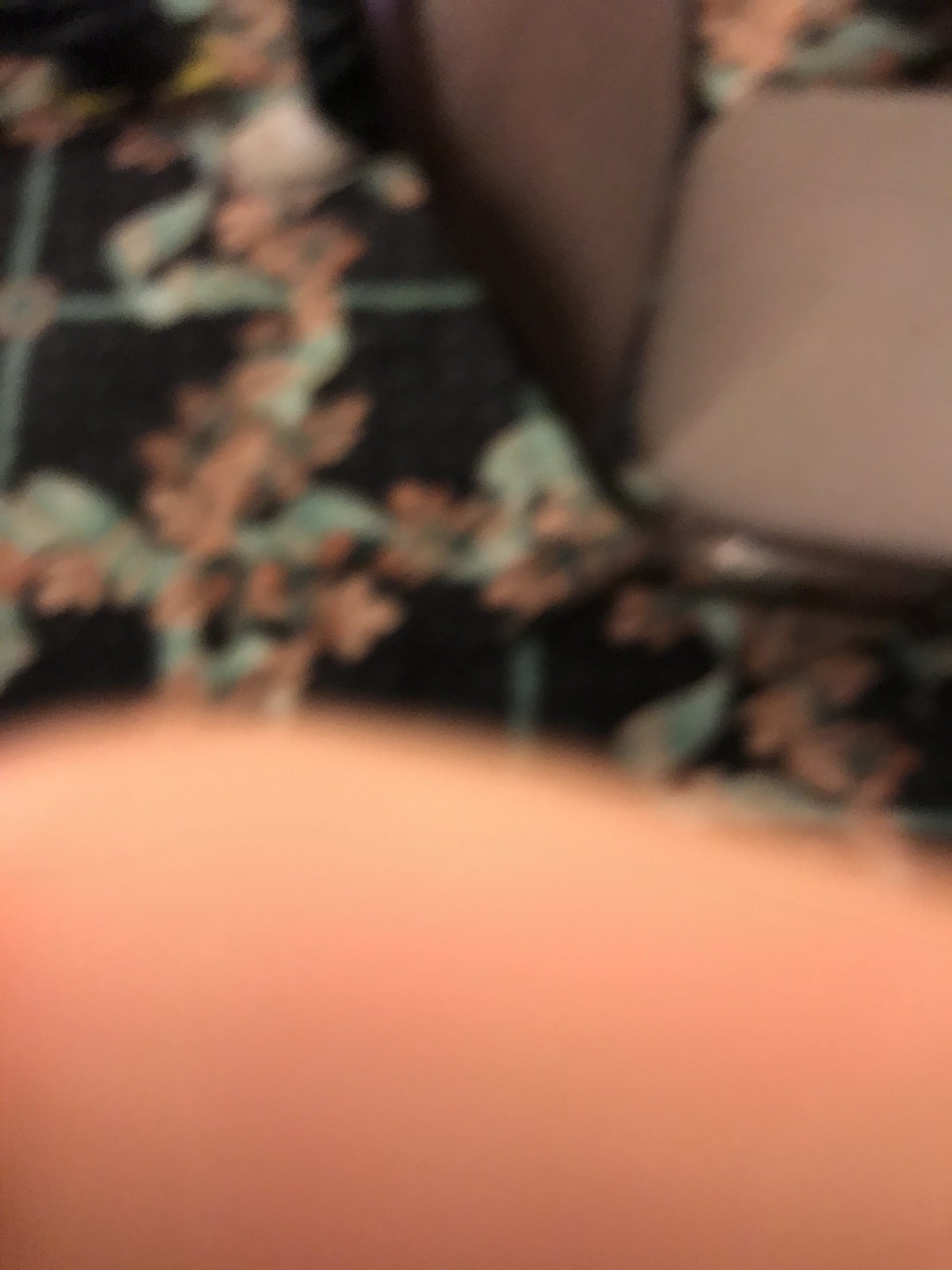In the foreground of this image, a blurred finger partially obscures the view, occupying the bottom third of the picture. In the background, a tan-brown chair with black outlined details is visible. The image's main focus, however, is the intricate floor design beneath both the chair and the finger. The flooring features a black base with blue-outlined squares, each containing a floral print. The floral patterns within the squares combine blue and pink hues; the vertical elements predominantly showcase pink tones, while the horizontal elements display a more intricate mix of blue and pink shades. This detailed arrangement creates a visually engaging and colorful backdrop.